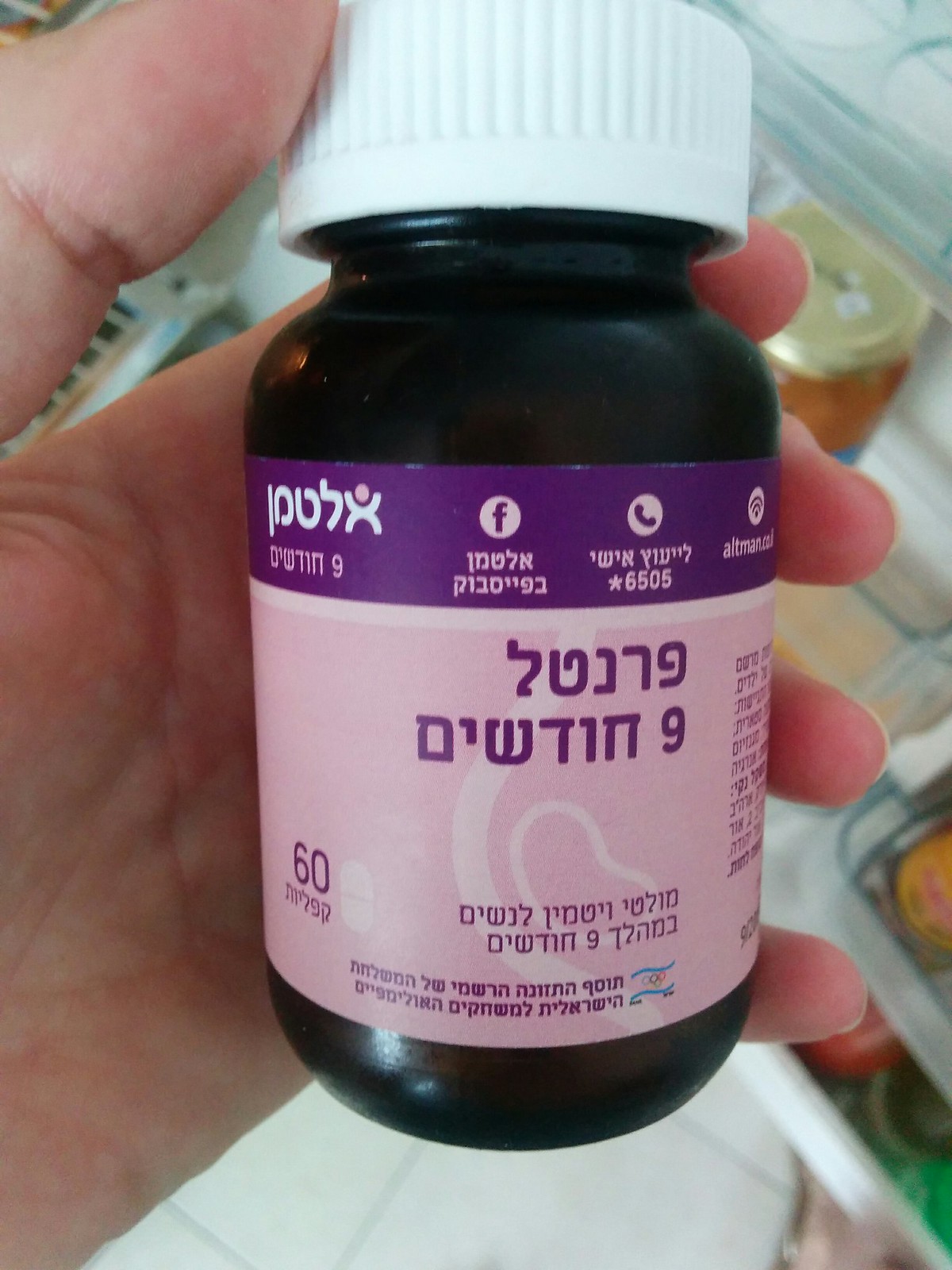The color photograph, captured in portrait orientation, focuses on a dark brown, almost black, opaque glass medicine bottle held by a left hand. The hand, cut off just above the thumb, shows the thumb pointing diagonally upward from the top left while the fingers curl around the bottle on the right. The bottle is equipped with a recognizable ribbed white cap, typically requiring a press-and-twist action to open. Encircling the bottle is a distinctive label: the lower portion features a pink background, while the top section is adorned with a dark purple strip. The label includes several white icons including a Facebook logo, a telephone icon, and a Wi-Fi symbol. Amidst the purple text on the label are Hebrew characters, and prominently on the left side near the back there is the number "60" indicating the likely quantity of tablets or pills inside. Additionally, other text on the label, such as "altman.co.nni", hints at website or contact information. The bottle’s contents remain obscured due to the opacity of the glass.